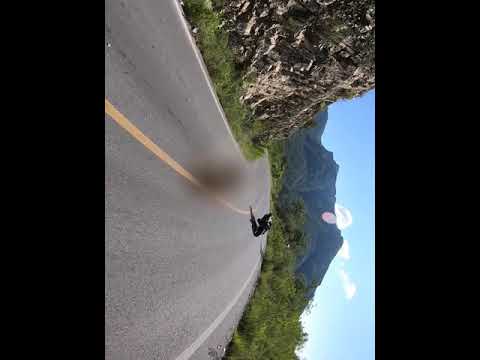In this dynamic photograph captured from the viewpoint of a motorcyclist, we see a scenic road scene that emphasizes the thrill of the open road. The image is rotated, providing a unique, sideways perspective. Dominating the foreground is a well-maintained, two-lane gray asphalt road with a prominent yellow line running through its center, framed by white stripes on each side. Leaning heavily into a turn at the center of the image is a motorcyclist dressed in black and white, riding a sleek black motorcycle. The left side of the image features a cliffside adorned with rugged white and tan rocks, while the right side showcases lush green vegetation and trees. In the distance, a majestic mountain covered in verdant greenery rises against the backdrop of a light blue sky adorned with a single white cloud. The entire scene is bathed in the sunlight of a clear day, perfectly capturing the essence of an adventurous ride through a picturesque landscape.